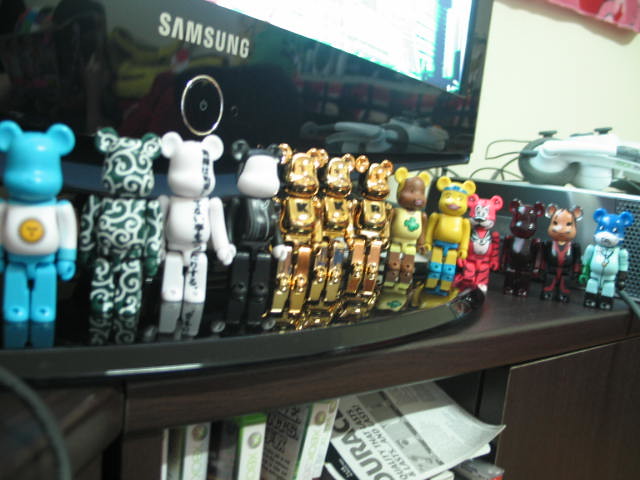The photograph captures a meticulously arranged collection on a TV stand, centered around a modern Samsung TV. The TV, characterized by a black frame with a touch-sensitive circle and a reflective surface, dominates the middle of the frame. The surface below the TV reflects the room's lower portion and emits a white light. A display of video games and a gaming console, possibly an Xbox, is also visible.

Surrounding the TV are numerous small, upright figures, all modeled after the same mouse character but featuring different skins. Some mice are entirely blue with white shirts, while others are all white, some with Asian-inspired patterns. The collection includes three golden mice, one yellow mouse, and one dressed in a tiger suit. Although initially mistaken for bears, the figures are, in fact, uniform in size and posture, each uniquely adorned, including variations resembling superheroes, nurses, and businessmen. The figures contribute to the whimsical and diverse aesthetic of the display.